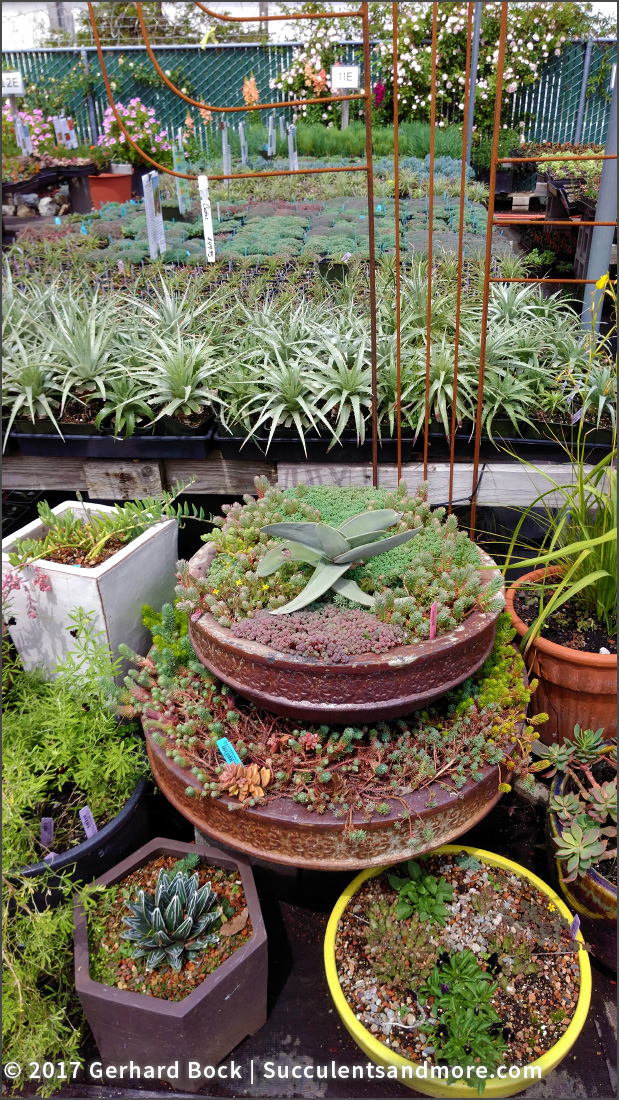This outdoor photograph captures a bustling plant nursery specializing in succulents and other greenery. The foreground is dominated by various raised planters – round, hexagonal, and square – filled with different types of succulent and foliage plants. A notable feature is a prominent multi-layered water fountain-like display overflowing with diverse greenery, including cactus and aloe vera, which adds a unique aesthetic to the scene. Adjacent to this arrangement stands a copper-colored metal trellis that visually separates the foreground planters from the raised tables in the background. These tables are laden with black plant trays hosting spiky green succulents and a stunning array of mixed greens. The far background is dotted with a sparse smattering of small pink and white flowers, providing subtle color accents. The bottom of the image bears the text "2017 Gerhard Bach Succulents and More," indicating the commercial context of the display – likely part of a garden shop or garden center exhibit. The overall scene is rich in varying shades of green, from light to dark, highlighting the diversity and lushness of the plants on display.